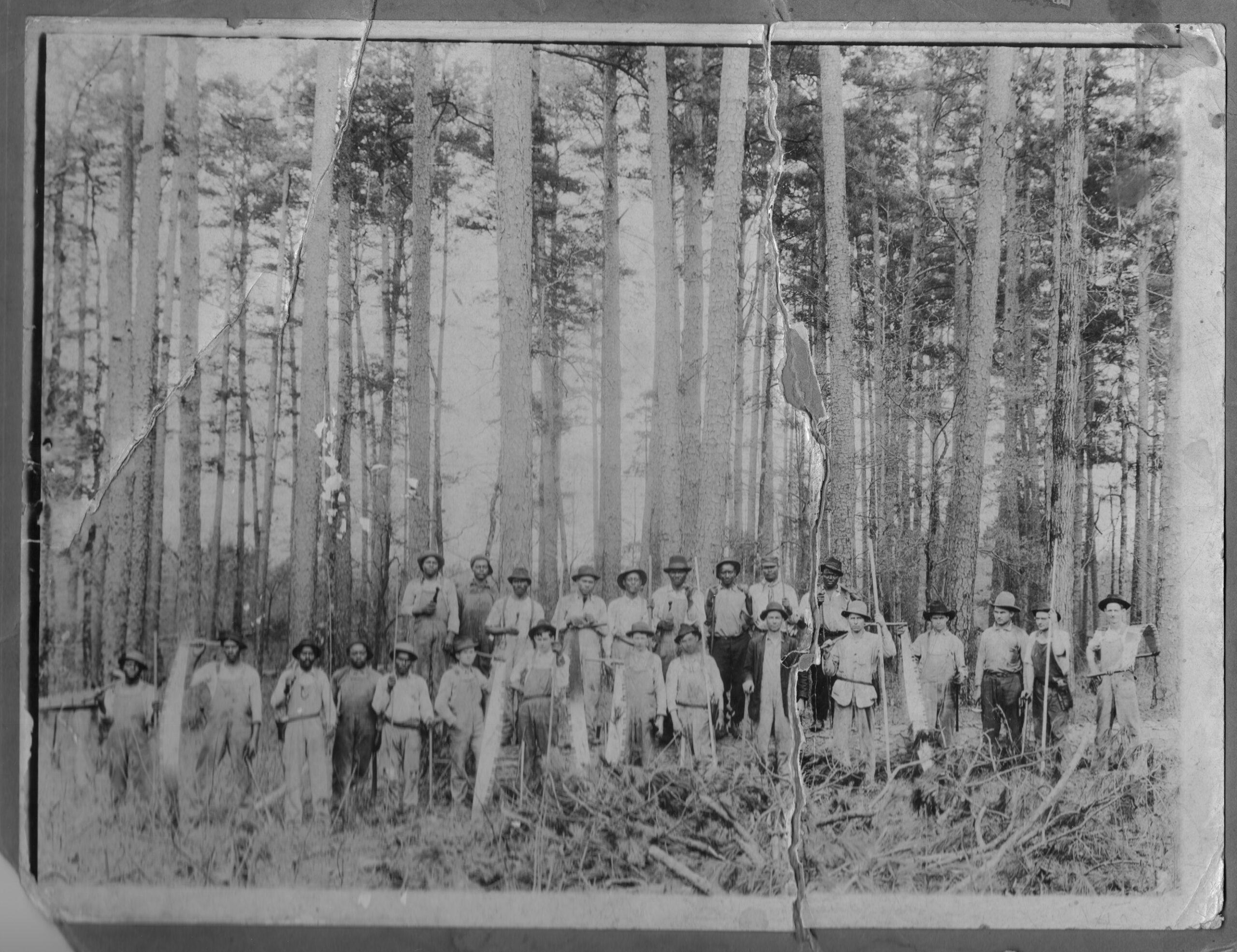This image is a damaged black and white photograph from the 1800s, depicting a large group of approximately 30 men standing in two rows in a clearing surrounded by tall trees. The photograph shows signs of age, with visible wrinkles, folds, and tears that have seemingly been taped together. Most men in the photograph appear to be African American, with a few white men also present. They are all wearing hats and work clothes, predominantly overalls. The men are equipped with large hand saws, the type used by teams to cut down trees, indicating that they are lumberjacks. The overall scene captures these workers amidst a forested background, suggesting a lumberjack team's photograph from the era.